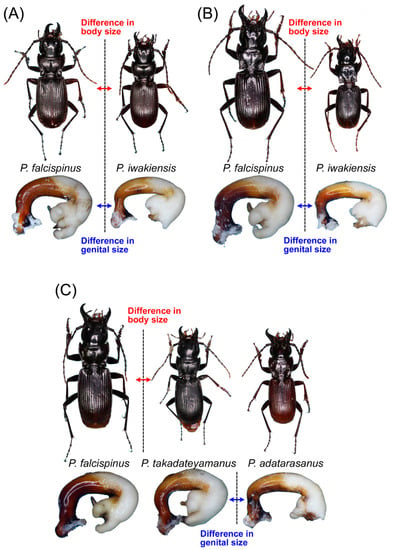This image features a detailed diagram on a white background comparing three different stag beetles, labeled A, B, and C. Each section highlights both body size and genital size differences among the beetles, with clear labels indicating "Differences in body size" in red and "Differences in genital size" in blue. Diagram A compares P. falcispinus with P. awakinsis, illustrating their varying body and genital sizes. Diagram B continues this comparison between the same two species, emphasizing similar distinctions. Finally, Diagram C introduces P. tachydateaemanus and P. adataresanus, in addition to P. falcispinus, further showcasing variations in body and genital sizes among these stag beetles. The beetles are depicted in black, with annotations and measurements providing a thorough comparison of their anatomical differences.